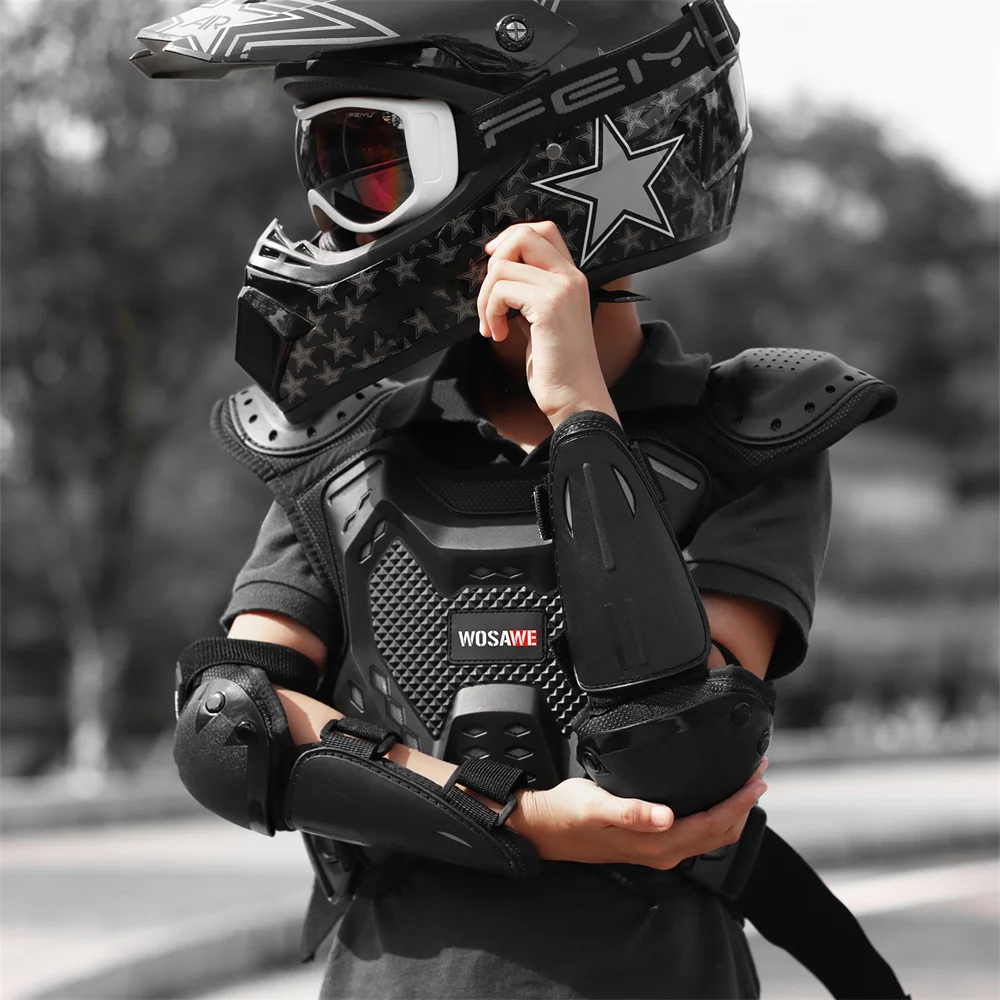The image features a person dressed in padded motorcycle gear, standing against a grey background with blurred elements including trees, creating a black-and-white contrast against the color-rich subject. The individual is adorned in predominantly black attire with protective padding over their shoulders, elbows, forearms, and chest, marked with the logo "W.O.S.A.W.E" on the chest piece. They wear a black short-sleeve t-shirt underneath the armor. The helmet is a notable focal point: it's a large, black motorcycle helmet featuring multiple Dallas Cowboy stars, including a prominent larger star on the top and side. This helmet is complemented by red-lensed goggles with a white frame and a strap labeled "F.E.I.Y." The person's head is turned slightly to the right, although their body faces forward, and their hand is raised near their ear. This detailed composition suggests they could be a motocross athlete, given the robust safety gear and sporty appearance, though their petite frame hints they might be a young racer.